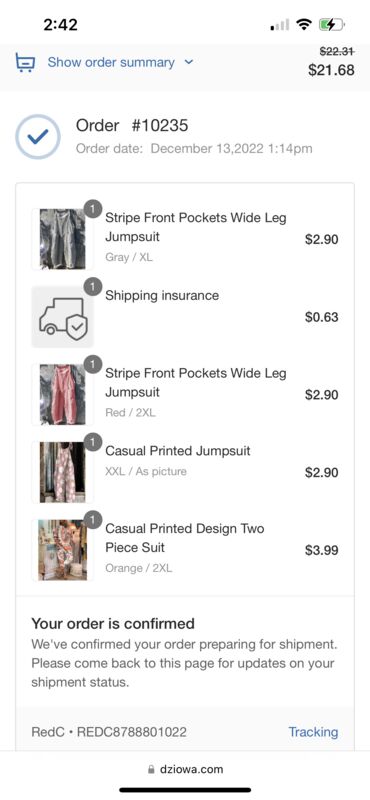**Order Confirmation - Clothing Site**

**Device: Mobile Phone**

- **Order Details:**
  - Total Amount: $21.68 (Discounted from $22.31)
  - Order Number: #10235
  - Order Date: December 13th, 2022, 1:14 PM
  - Battery Status: Less than half
  - Signal Strength: 1 out of 4 bars
  - Wi-Fi: Full connectivity

**Order Summary (Dropdown Menu):**
- **Blue Cart Icon:** Indicates "Show Order Summary"
- **Listed Prices:**
  - Original: $22.31 (Crossed out)
  - Final Price: $21.68 (Larger Font)

**Items Ordered:**
1. **Striped Front Pockets White Leg Jumpsuit**
   - Color: Gray
   - Size: XL
   - Price: $2.90
   - Quantity: 1
   
2. **Shipping Insurance**
   - Description: Graphic with a truck and badge
   - Price: $0.63
   - Quantity: 1
   
3. **Striped Front Pockets White Leg Jumpsuit**
   - Color: Red
   - Size: XXL
   - Price: $2.90
   - Quantity: 1
   
4. **Casual Printed Jumpsuit**
   - Size: XXL
   - Description: As pictured
   - Price: $2.90
   - Quantity: 1
   
5. **Casual Printed Design Two-piece Suit**
   - Color: Orange
   - Size: XXL
   - Price: $3.99
   - Quantity: 1

**Order Status:**
- **Your order is confirmed.**
- **We've confirmed your order and are preparing it for shipment.**
- **Check this page for updates on your shipment status.**
- **Tracking Information available:** DCIOWA.com